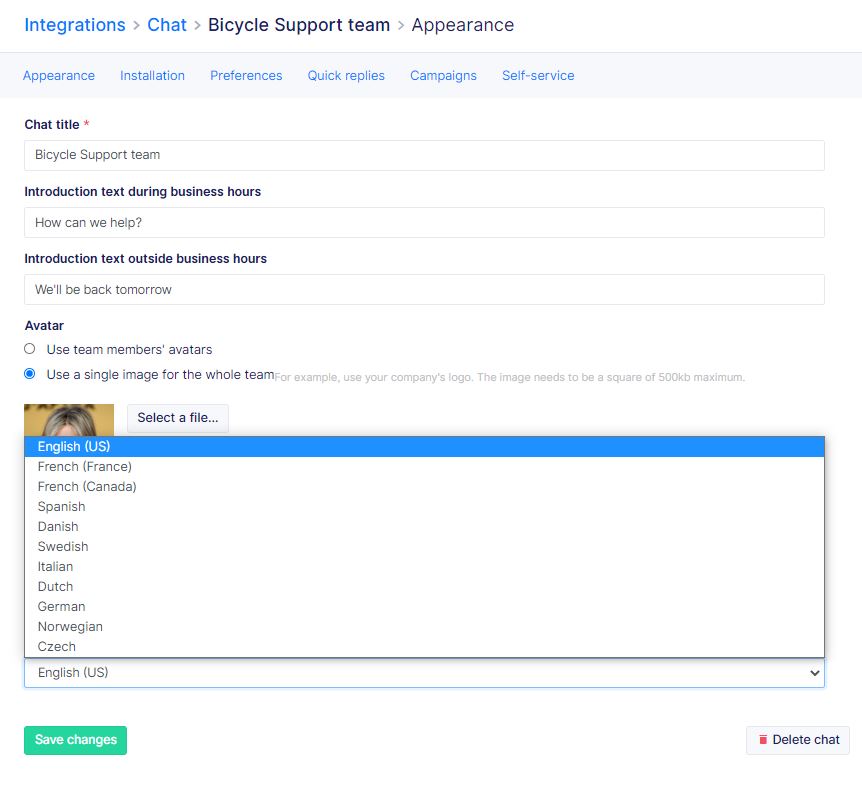The screenshot features a user interface with a white background. At the top of the interface, the words "Integration" and "Chat" are prominently displayed in blue. Below this header, a menu shows options titled "Bicycle," "Support Team," and "Appearance."

A light blue navigation bar spans the width of the screen just below these options, containing several clickable titles in blue: "Appearance," "Installation," "Preferences," "Quick Replies," "Campaigns," and "Self-Service."

Directly underneath the navigation bar, black text titles and a long white text box are visible for user input. Below this section, the word "Avatar" is displayed with two circle options next to it; the bottom circle is blue, indicating it has been selected. Adjacent to the avatar section, the upper portion of a profile picture is partially visible, alongside a gray button labeled "Select File."

The lower portion of the screen is partially obscured by a drop-down menu listing various languages, with "English (US)" highlighted but the menu not fully collapsed.

At the bottom left of the screen is a green button labeled "Save Changes," while the bottom right features a green button labeled "Delete Chat," accompanied by a small red square.

This layout suggests an editable form where users can input and modify information, switch languages, and manage their chat settings.